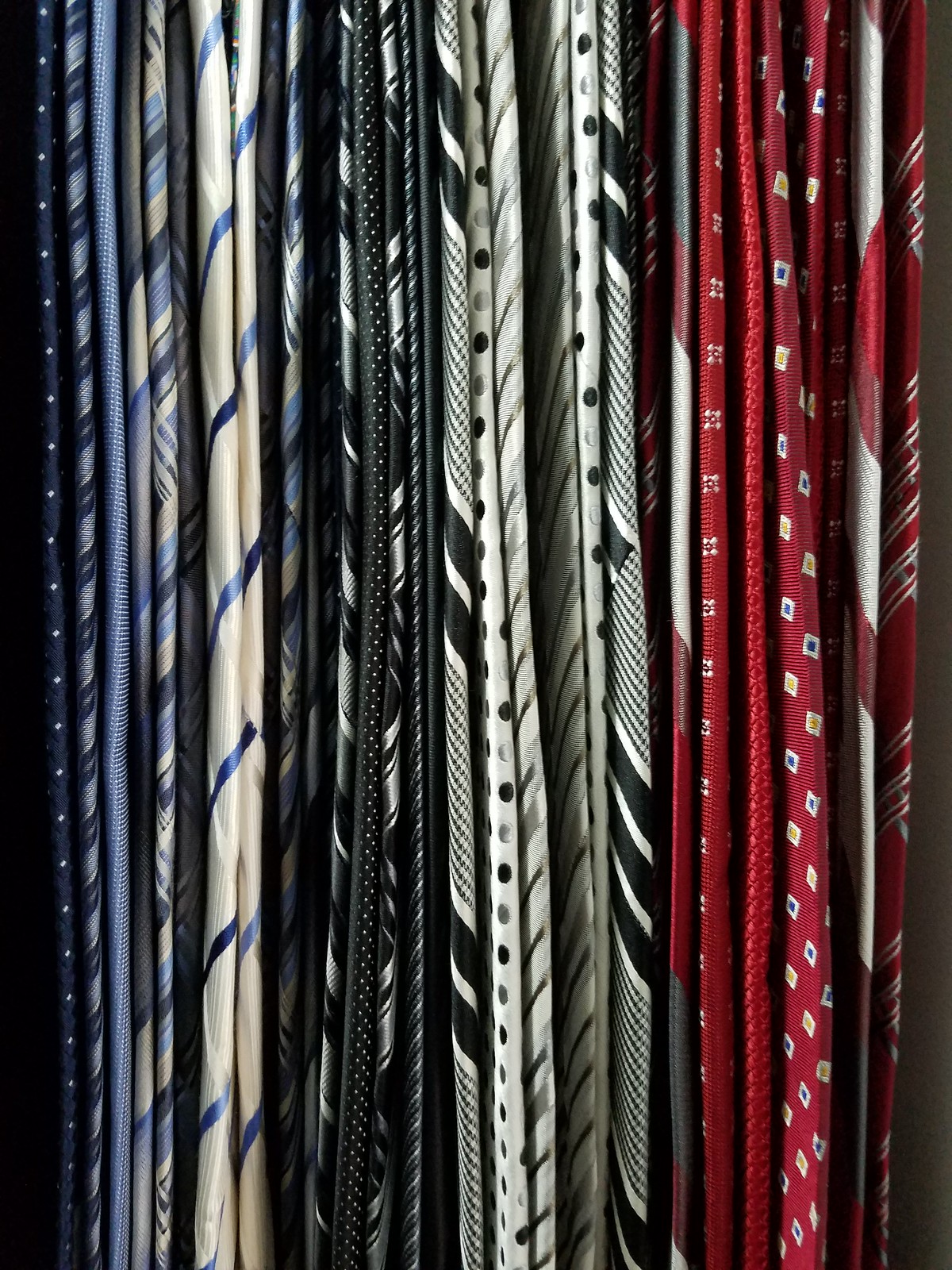The photograph captures a tightly packed array of over 20 different hanging neckties, neatly arranged in vertical rows. Starting from the left, the ties first present a spectrum of blues, including varieties with polka dots, stripes, patterns, and even a feathery texture. As the display progresses, the hues transition into a collection of blacks, featuring similar patterns of stripes, polka dots, and intricate designs. This is followed by a series of white ties, predominantly adorned with polka dots and striped patterns. Moving further to the right, the assortment culminates in a vivid array of red ties, showcasing checkered patterns, stripes, and other intricate designs. The ties span from navy blue on the far left through shades of blue, black, white, and finally to a deep crimson red on the far right. Despite the precise patterns on each tie, the overall image provides a striking visual display of predominantly blue, black, white, and red colors, suggesting they could be hanging on a tie rack, possibly in a shop or a closet, although the actual rack is not visible in the photo.